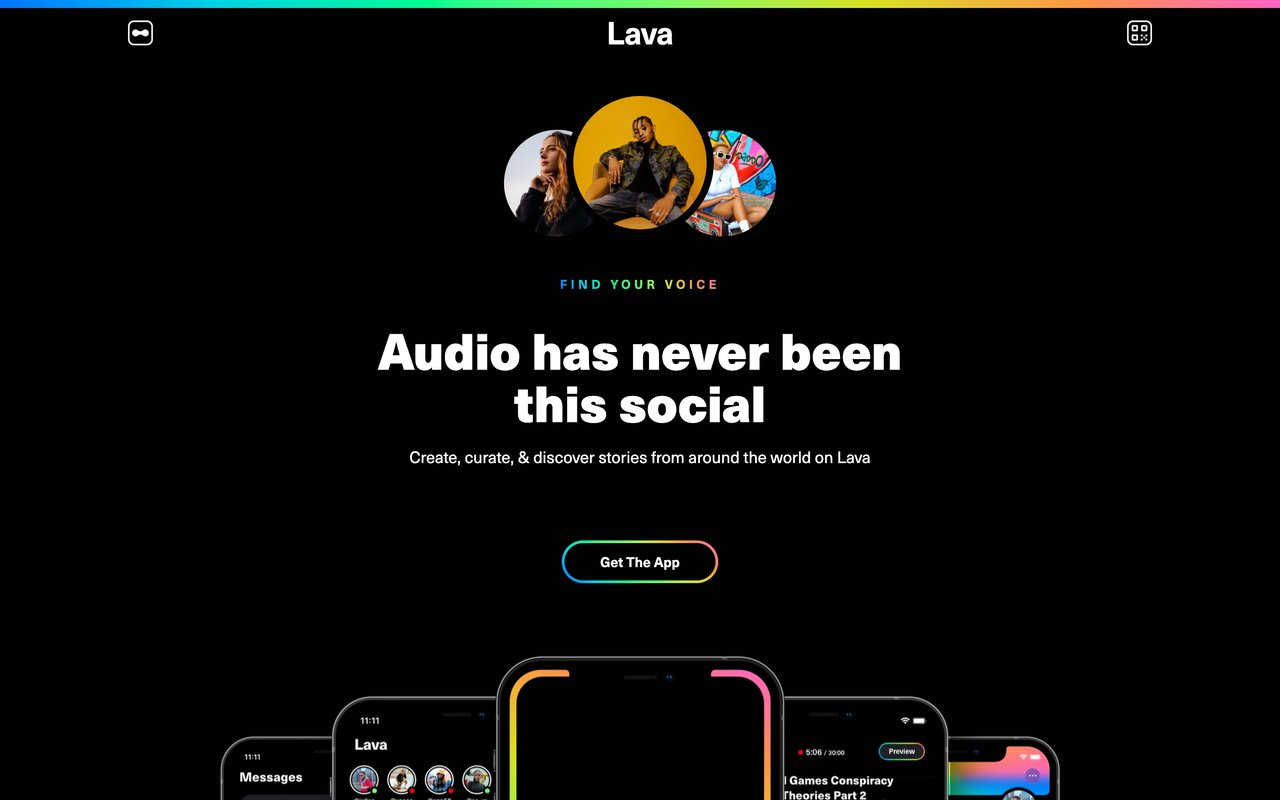The screenshot appears to depict a webpage for a social media-integrated audio platform known as Lava. The top section features a vibrant rainbow banner transitioning through various colors: blue, teal, green, light green, yellow, orange, and pink. 

In the upper left corner, there's a logo resembling two connected dots. The background is black, with the word "Lava" prominently displayed in the center. In the upper right corner, there are four small icons within a square.

Below the central "Lava" title, three circular profile images are showcased. The most prominent profile is a yellow-bordered circle featuring an African American male with braided hair, wearing a leather jacket and jeans, leaning back with a cool demeanor. Flanking him are two Caucasian women. The woman on the left, in a red-bordered circle, gazes off into the distance, while the woman on the right, set against a graffiti-painted wall, sports white sunglasses. Both women's images are slightly smaller and positioned behind the man's image.

Directly underneath this, a rainbow-gradient text reads "Find your voice," followed by a bold, large-font statement in white: "Audio has never been this social. Create, curate, and discover stories from around the world on Lava." Another call-to-action button prompts users to "Get the App," enclosed by a rainbow gradient border.

At the bottom of the page, a stack of five smartphones are arranged in a pyramid formation. The central phone is the most prominent, flanked by two phones on each side, positioned slightly behind and lower, creating a layered visual effect. These smartphones display various screenshots of the app, emphasizing its interactive and dynamic features.